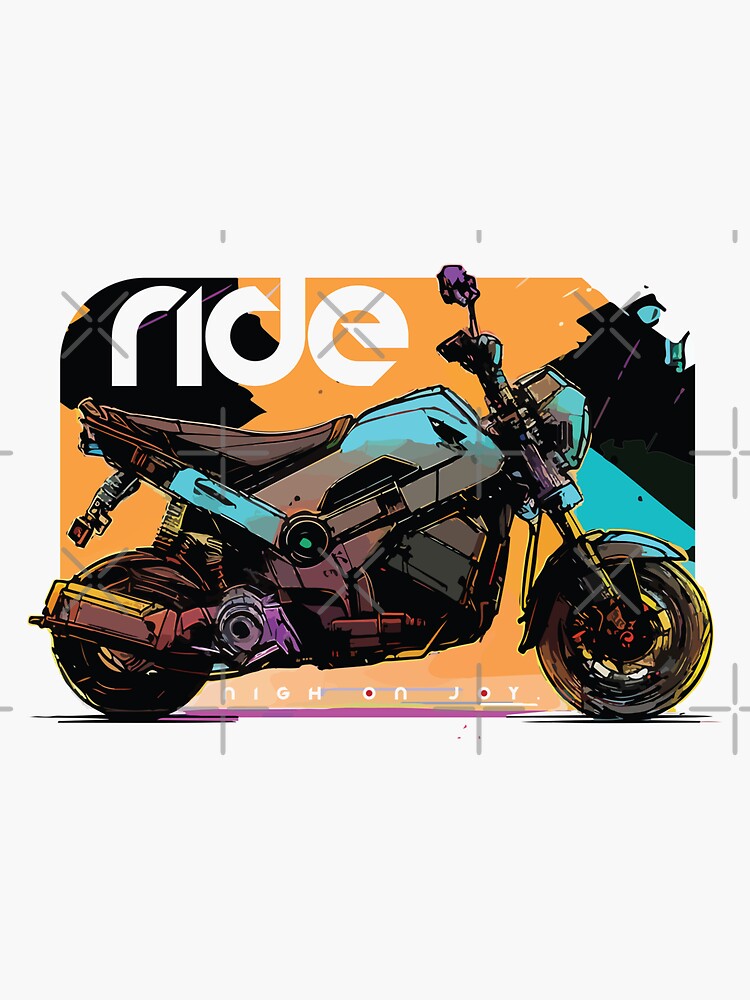This vibrant, cartoon-style digital artwork showcases a modernized, cyberpunk-inspired motorcycle against an eye-catching orange background. In the top left corner, the word "RIDE" is prominently displayed in large, rounded, white letters, with the "R" and "I" set against a black backdrop, and the "D" and "E" on the orange. The motorcycle itself is a striking amalgamation of colors: light blue fenders, yellow rims on the front wheel, and a predominantly black back wheel accented with metal rods. The sleek black seat is flanked by white rods. A purple streak underscores the bike, adding movement to the composition. At the bottom, the phrase "HIGH ON JOY" appears in smaller white letters on the same vibrant orange background, encapsulating the exuberant and playful essence of the piece. Subtle gray plus signs, acting as a watermark, are scattered across the image, adding to its textured, layered look. A delicate purple flower, possibly tied to the handle, adds a final touch of whimsy.